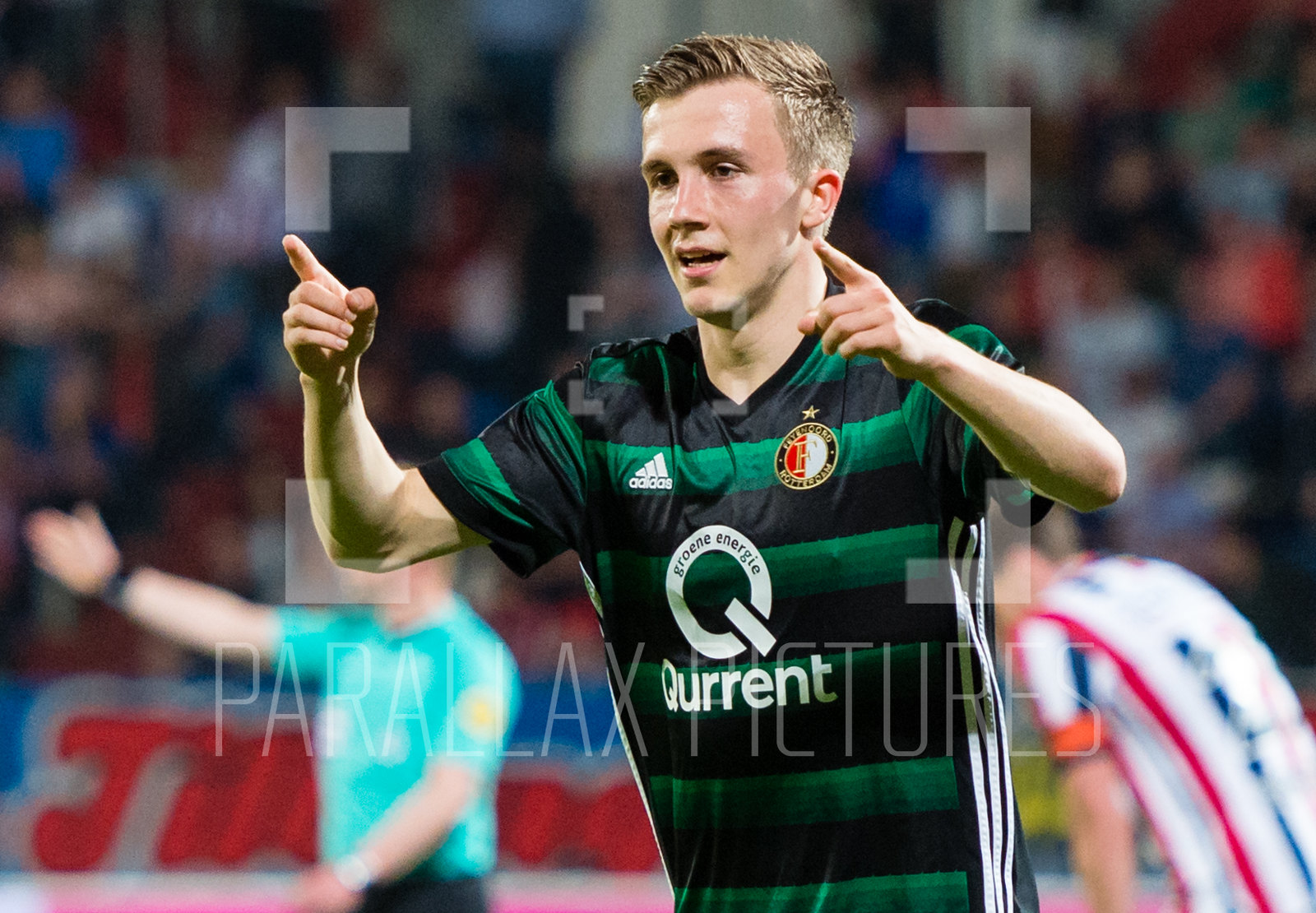This rectangular photograph captures the dynamic scene of a soccer player in the midst of a spirited celebration on the field. The central figure, a Caucasian man with short hair and dark eyes, is vividly depicted with his mouth open and both hands raised, index fingers pointing, exuding enthusiasm. He dons a green and black striped jersey emblazoned with "Grillon Energy Current," a "Q" emblem, and the Adidas logo visible on the right edge. The background is intentionally blurred, highlighting other indistinct players, including a nearby player in a red, white, and blue striped jersey bent over, and another figure possibly a referee in a teal shirt with dark pants, all set against a backdrop of fans in the stands. The bottom of the image features a watermark that reads "Para Parallax Pictures."